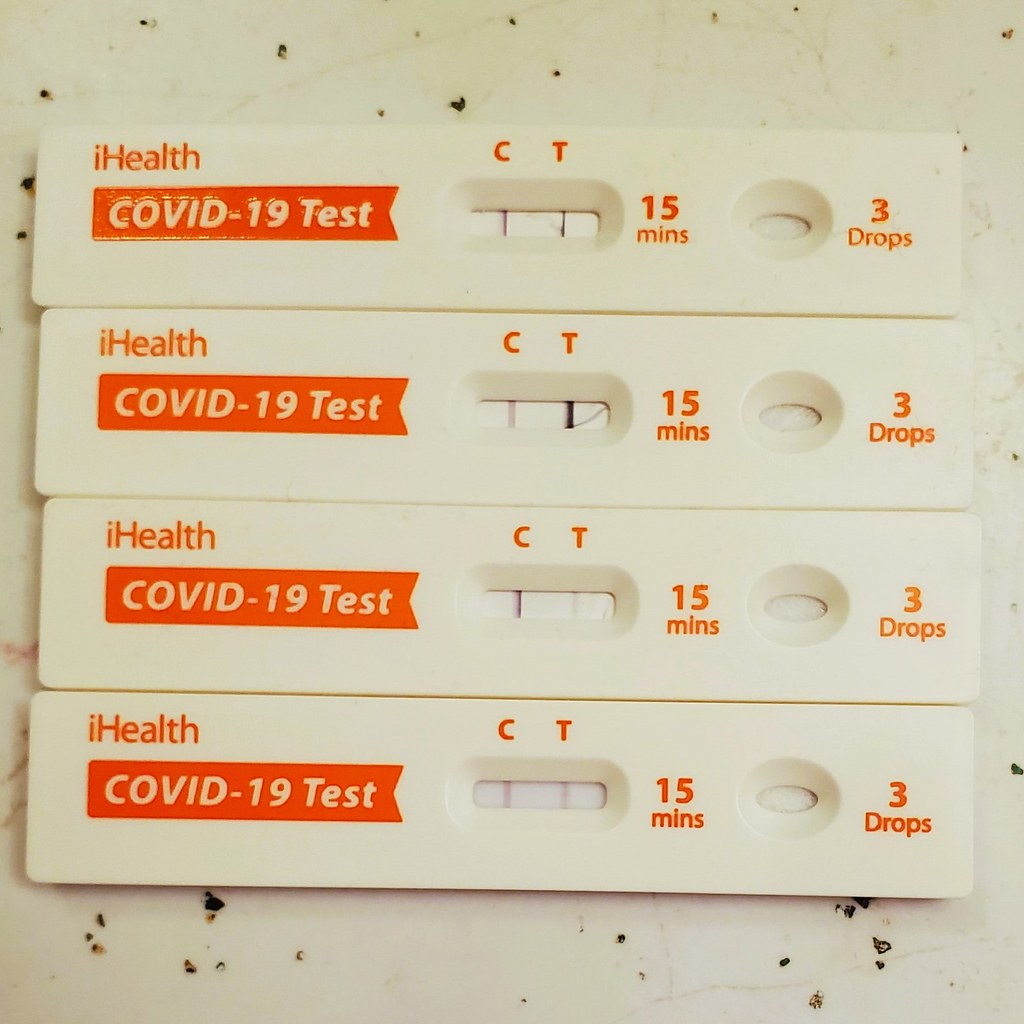This overhead photo captures four used COVID-19 test kits arranged side by side on a flat surface. Each kit consists of a white plastic strip featuring an indicator window with the "C" and "T" markers and a designated area for three drops. Labels on the left side of each kit read "Eye Health," followed by "COVID-19 Test" against a reverse red background. The instruction to place three drops is prominently displayed along with a "15 minutes" timer. The indicator windows on the kits show varying results. The kits are placed on a white countertop speckled with black, irregular patterns, providing a clear and contrasting background. The uniform arrangement of the white test kits against the speckled surface forms a tidy and focused composition within the square frame of the photo.